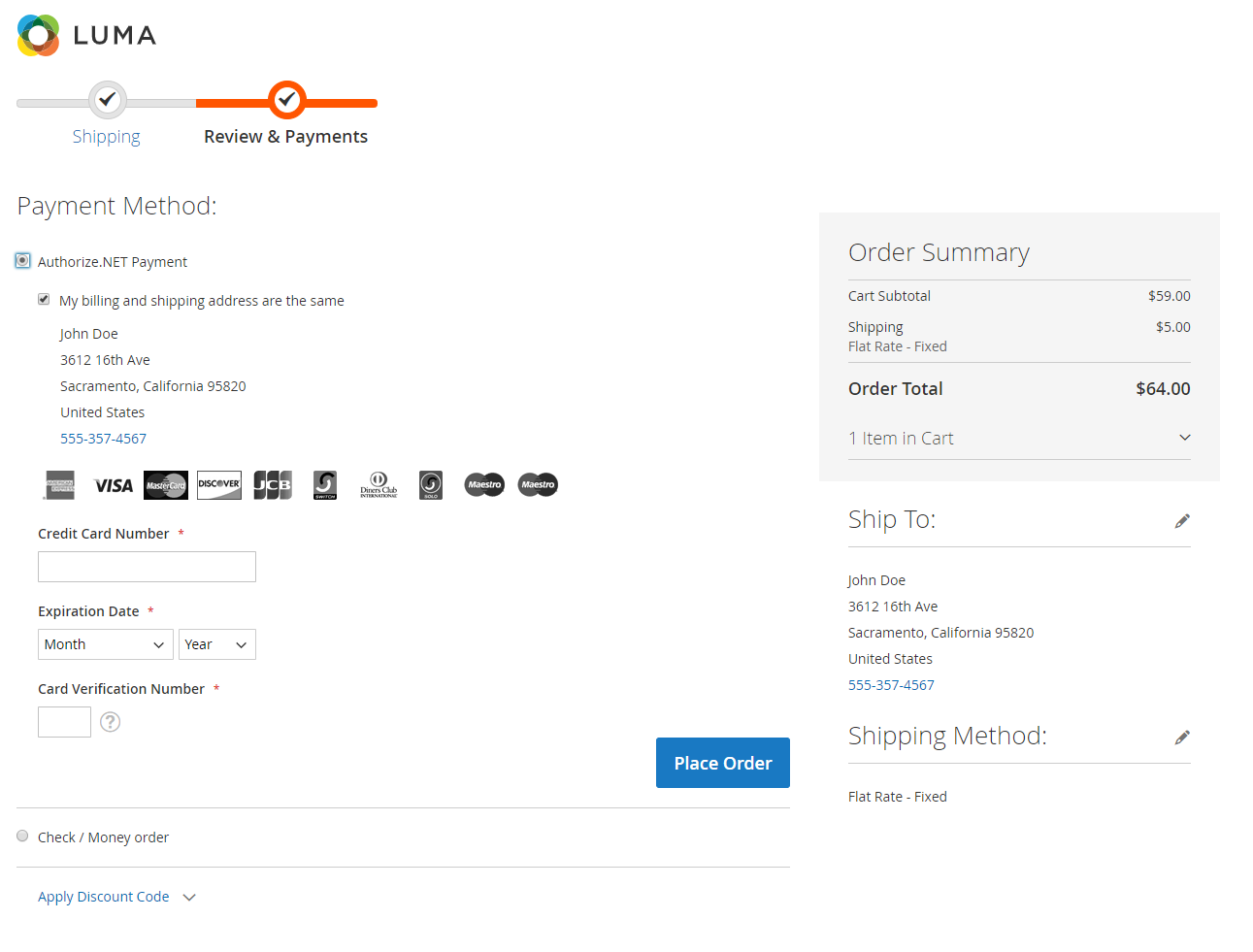In the upper left corner of the image, there is a circular emblem divided into four color segments: blue, green, orange, and yellow. Beside this emblem, the word "LUMA" is prominently displayed in bold, uppercase letters. Beneath this, a gray line passes through the middle of the circle, with the word "Shipping" written in blue below it. 

Continuing downward, an orange line leads to an orange circle positioned at the center, containing a check mark. Directly beneath this are the words "Review and Payments" in black. Below this heading, the term "Payment Method" appears with "Authorize.net Payment" following it. In smaller text, it states, "My billing and shipping addresses are the same," followed by "John Doe, 3612 16th Avenue, Sacramento, California, 95820, United States," with the phone number "555-357-4567" in blue. 

In the top right corner, a blue box contains the text "Place Order" inside a gray box. An order summary is also located in the upper right corner, detailing the cart subtotal, listed as "$59" to the left, with "Shipping Flat Rate Fixed" shown as "$5" to the right. The order total is clearly displayed as "$64" around three inches over.

Additionally, the image indicates that there is "1 Item in Cart." At the bottom right corner, the shipping method is labeled "Flat Rate Fixed."